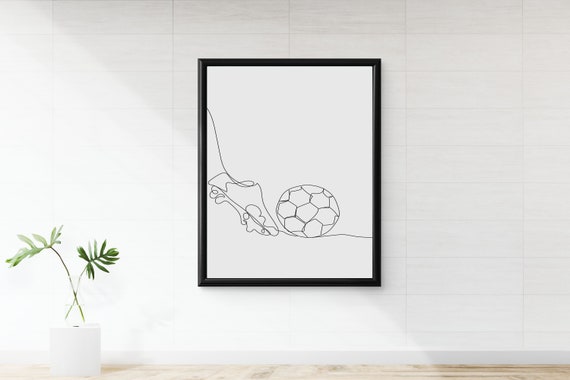The image showcases a detailed scene with a white wall as the background. Prominently displayed in the middle of the wall is a large, black-framed artwork that features an abstract black and white line drawing. The drawing appears to depict a soccer ball with distinct hexagonal patterns on the right side, and what resembles a shoe on the left, with lines extending from the top left corner towards the bottom right, adding to the abstract quality of the image. Below, on a light brown wooden floor, there's a white planter on the bottom left corner containing two green leaves or stems, which cross each other in an X shape. The plants have broad leaves and a spiky appearance, contributing to the overall artistic setup.